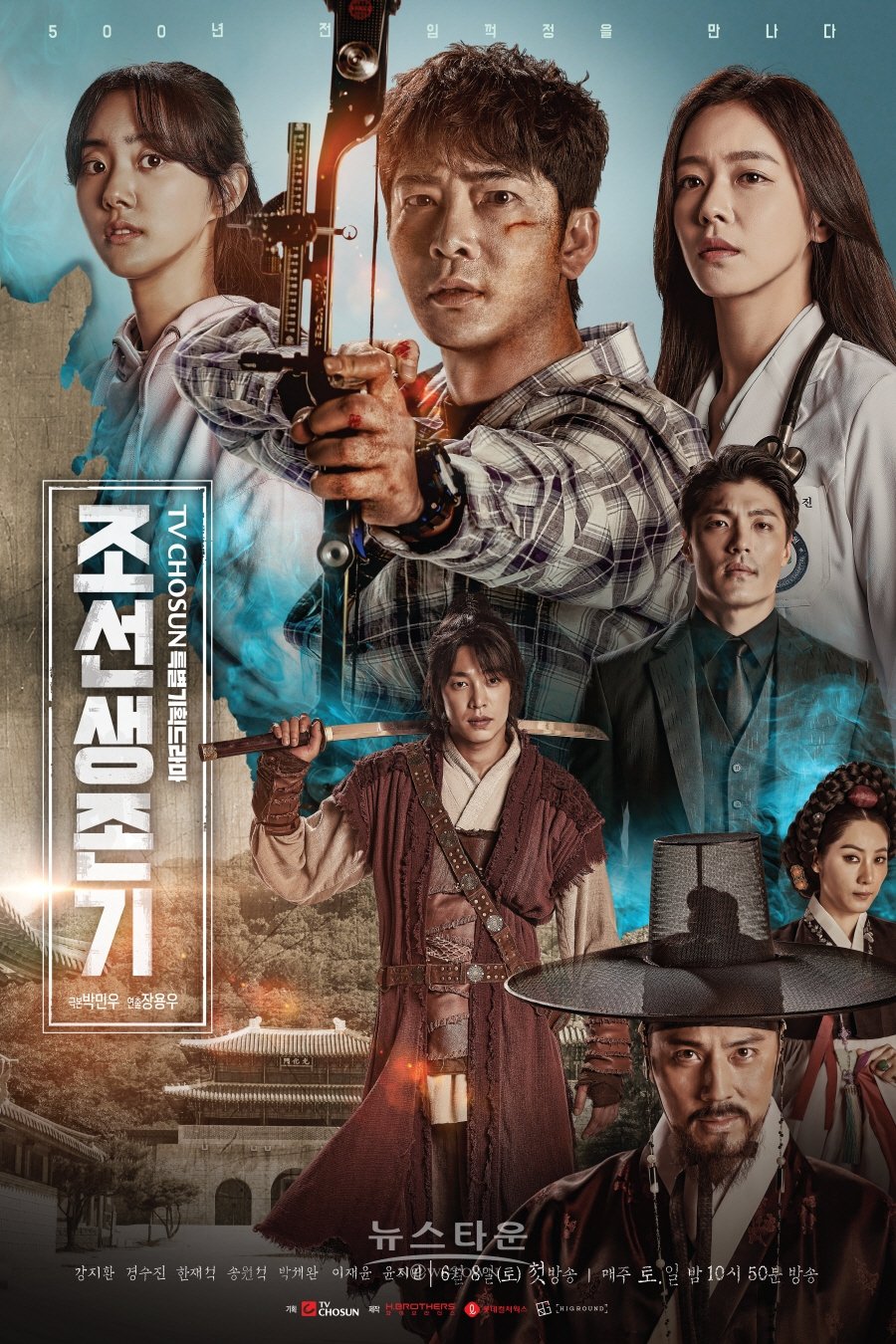In this movie poster, the title is displayed at the very top in white letters that are not in English. The central focus features seven characters. The top row showcases the three tallest figures: starting from the left, a woman wearing a gray sweatshirt with a blue light accent at the bottom; in the middle, a man in a gray and dark gray checkered shirt holding a bow in front of him; and on the right, another woman wearing a white jacket with a stethoscope draped over her shoulder.

Below them, from left to right, there is a man dressed in a black suit with short black hair, a person in a brown robe holding a sword behind her head, a man in the bottom right corner wearing a black hat, and a woman beside him dressed like a maid.

The left side of the poster features Asian characters, along with the number "71." The background includes a large, structured building on the left and a lush display of green leaves.